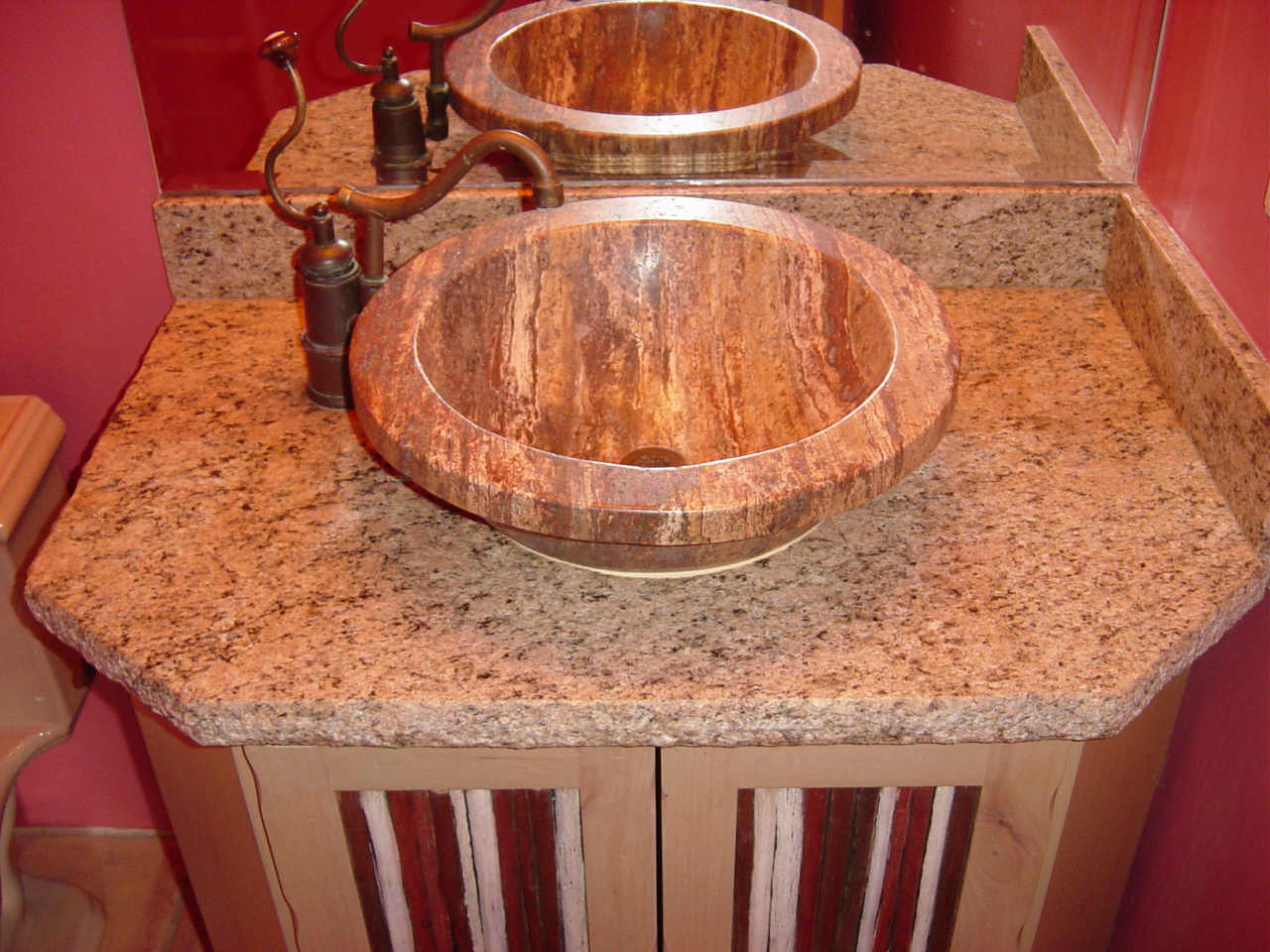The photorealistic image showcases a bathroom sink that exudes vintage charm with its old-fashioned design. The countertop is crafted from traditional granite, providing a sturdy and elegant base. The sink itself is a unique wooden basin, evoking a classical or medieval aesthetic yet still maintaining high quality. The rustic copper faucet complements the basin, featuring a complex structure with a base, lever, and a winding pipe from which water flows. A mirror in the background captures the reflection of the sink and faucet lever, adding depth to the scene. To the left, a glimpse of a toilet seat and bowl is visible. The bathroom's backdrop is painted in a muted pink, enhancing the vintage feel. Beneath the sink, there is a two-door cabinet in brown, with only the tops visible as the handles are obscured. At the center forefront, a rectangular object with alternating red and white vertical stripes stands out, its uneven numbering adding an intriguing visual element.